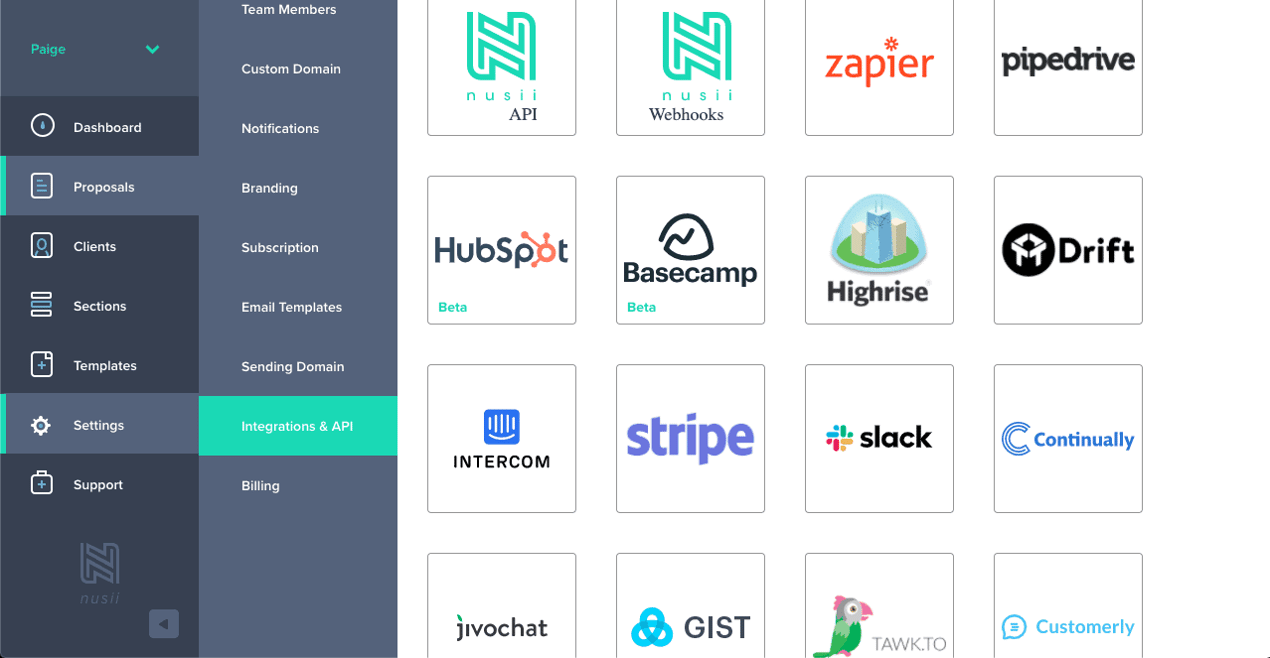This screenshot displays a structured interface from the Nusty application, showcasing various sections and integration options. On the left sidebar, there is a vertical menu with a drop-down arrow labelled "Page." Below this, the menu lists several primary sections: Dashboard, Proposals, Clients, Sections, Templates, Settings, and Support. Underneath these options, there is an "N" icon next to the text "Nusty" and a back arrow.

Further down the sidebar, additional menu options include: Invite Team Members, Custom Domain, Notifications, Branding, Subscription, Email Templates, Sending Domain, Integrations and API (which is highlighted in green), and Billing.

The main section of the screenshot is organized into a 4x4 grid, presenting various integration options available within the Nusty system. These integrations include:

1. Nusty API
2. Nusty Webhooks
3. Zapier
4. Pipedrive

5. HubSpot
6. Basecamp
7. Highrise
8. Drift

9. Intercom
10. Stripe
11. Slack
12. Continually

13. JivoChat
14. Gist
15. Talk.to
16. Custom Early

This detailed organization allows users to efficiently navigate through different functionalities and integrations within the Nusty platform.